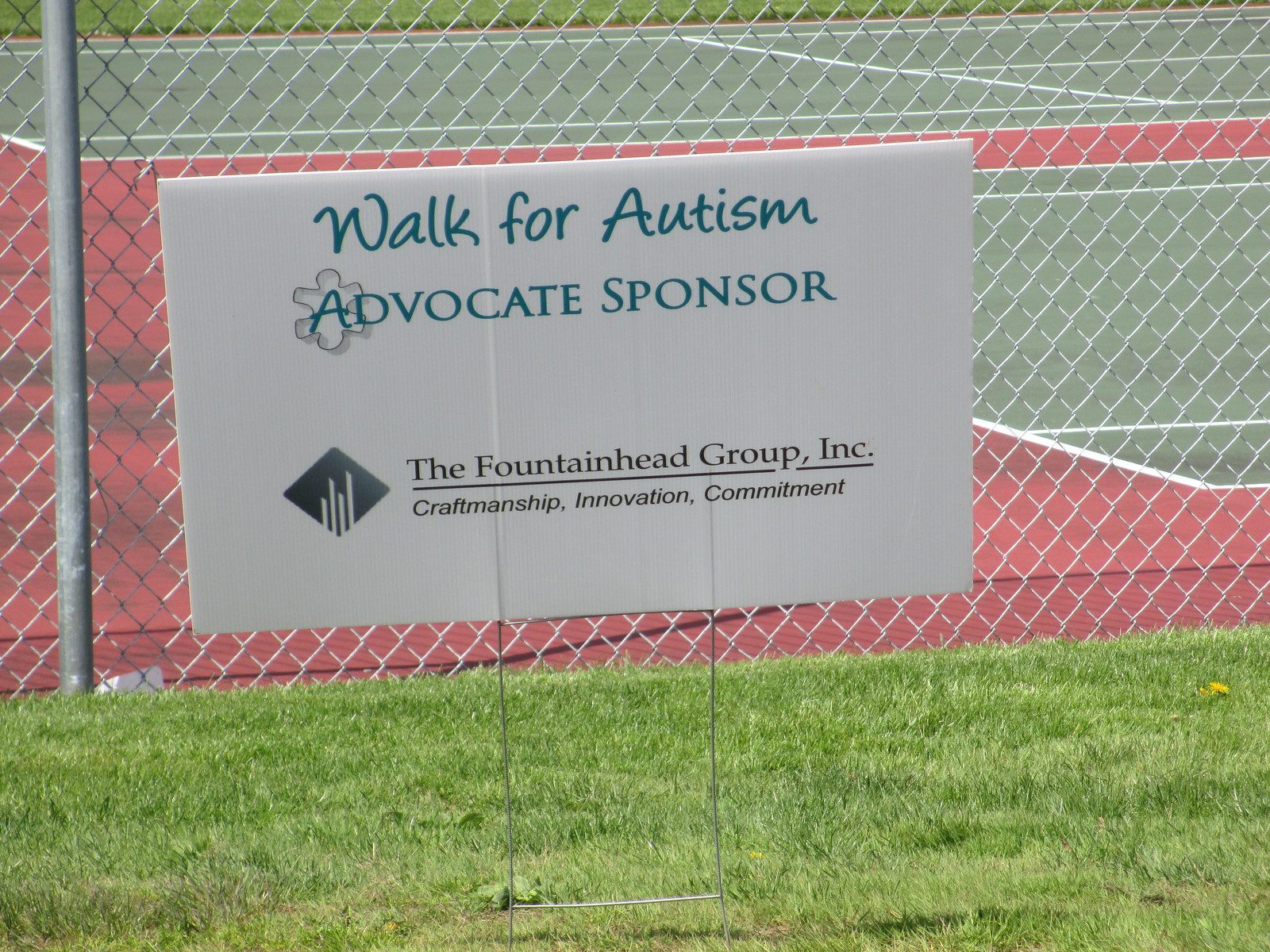This image captures a meticulously maintained, bright green grassy area with a prominently displayed white sign as its focal point. The sign, held upright by thin metal stands, reads in turquoise lettering, "Walk for Autism, Advocate Sponsor." Below that, in black font, it states, "The Fountainhead Group Incorporated" accompanied by their slogan, "Craftsmanship, Innovation, Commitment." The logo of the Fountainhead Group is black and diamond-shaped with intersecting lines.

Positioned in front of a silver metal gate with a diamond-patterned chain-link, the sign stands at the edge of the grassy surface. Stretching beyond the gate are two tennis courts with a distinctive red clay separation area and green playing surfaces marked by white lines. The absence of people in the scene emphasizes the tranquility of this outdoor setting, under a clear sky, showcasing the purpose of the sign for an autism fundraising event without any obstructions.